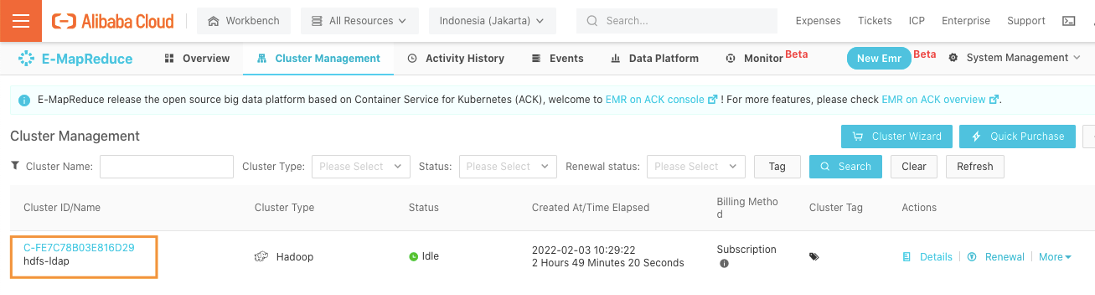The image depicts a user interface for Alibaba Cloud's Workbench, specifically focusing on resources in Indonesia, Jakarta. 

At the top left, the "Alibaba Cloud" logo is displayed in orange, followed by the title "Workbench, All Resources in Indonesia, Jakarta." To the right, there is a search box for easy navigation. Adjacent to this are the options "Expenses," "Tickets," "ICP," and "Enterprise Support."

Below this section, there are several navigational tabs including "EMAP Reduce," "Overview," "Cluster Management" which is highlighted in blue, "Activity History," "Events," "Data Platform," and "Monitor," the latter of which is marked as being in beta with red text.

A blue button labeled "New EMR" also features a red "beta" tag next to it. A gear icon indicating "System Management" is situated beneath this.

Further down, a description reads: "EMAP Reduce, Release the open-source big data platform based on container service for Kubernetes (ACK). Welcome to EMR on ACK console. For more features please check EMR on ACK overview."

The interface then focuses on "Cluster Management," displaying fields such as Cluster Wizard and Quick Purchase, both represented as blue buttons. A field labeled "Customer Name/ID/Name" followed by an identifier "C-FE7C78B03E816D29" is highlighted in an orange box, indicating its selection or importance in the context.